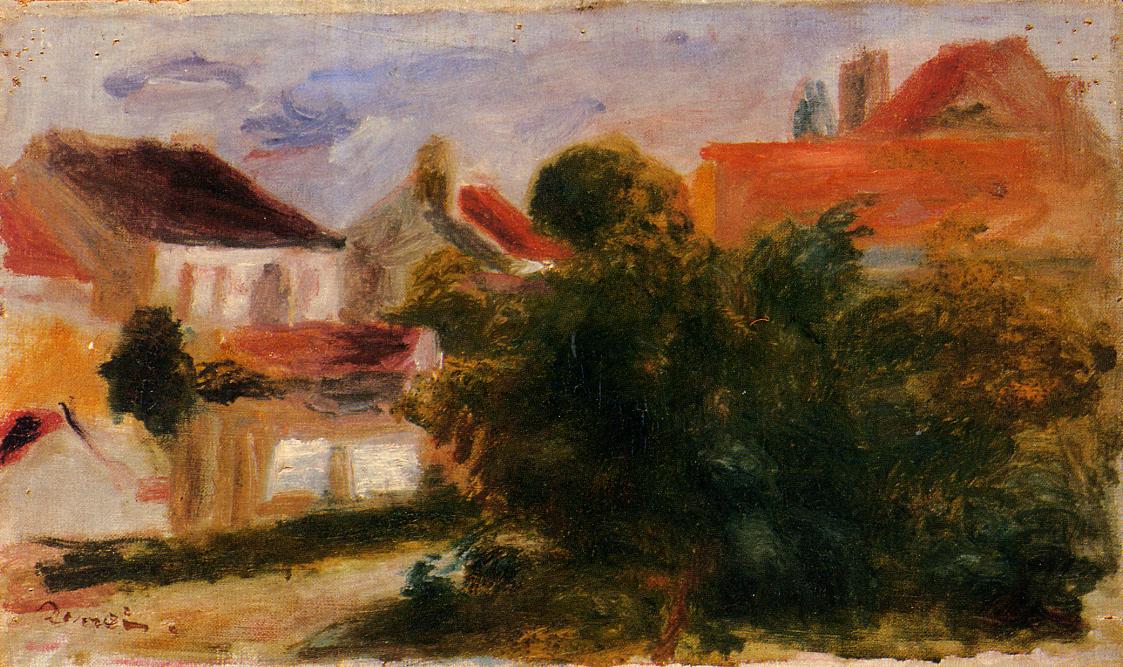The painting is a vibrant and textural rendition of a townscape, evocative of Van Gogh's impressionistic style. The top third of the image is dominated by a light grayish-blue sky with hints of white clouds, suggesting the sun is just below the horizon, casting a soft, ethereal light. The foreground to the right features what appears to be a green space, possibly dense bushes or a small forest, adding a natural, earthy touch. Nestled among the greenery, one can glimpse a building with an orange roof and a tall, brown tower behind it. 

The left side of the painting shows several houses with a distinctive, pinkish-gray facade and dark rooftops, further contributing to the earthy tones. One house, in particular, stands out with its white front and dark roof. Between these prominent structures, various other buildings can be discerned through their windows, though they remain somewhat obscured and unfocused. 

The overall palette is rich and varied, incorporating shades of red, blue, green, and sandy hues, giving the scene a lively yet somewhat muted atmosphere. This blend of colors and textures creates a vivid but abstract representation of the townscape, emphasizing the artistic complexity and emotional depth. Notably, the scene is devoid of any human figures, focusing entirely on the interplay of architectural and natural elements. An unreadable artist's signature, potentially "Renard," is located in the lower left, adding a subtle, personal touch to the artwork.